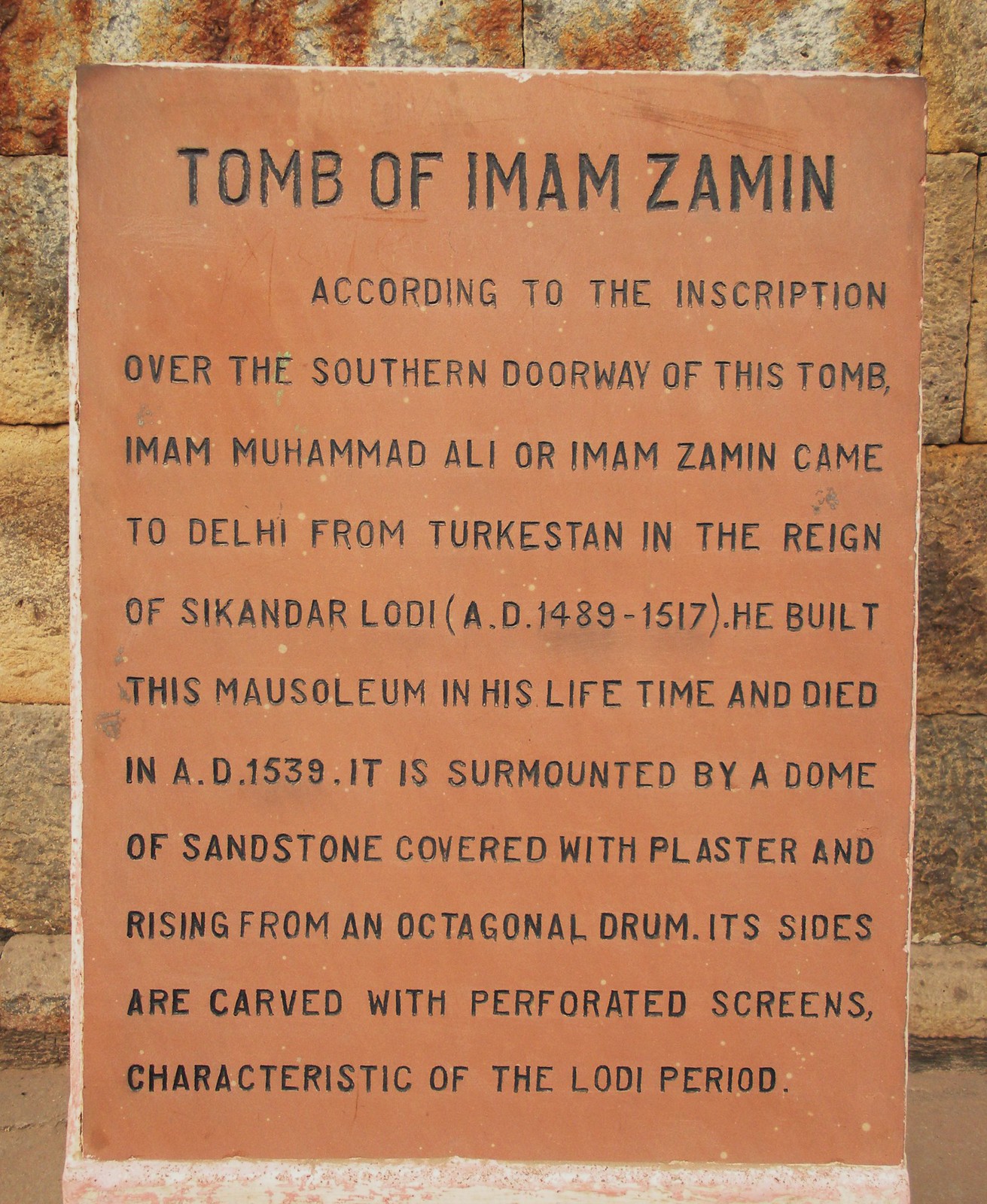The image features a prominently displayed reddish-brown stone or clay plaque, intricately inscribed with capital black letters. This plaque is either embedded into, leaning against, or standing in front of a brick wall, which exhibits shades of red, brown, and yellow. The plaque bears the inscription: "Tomb of Imam Zamin." Below that, detailed text recounts the history of Imam Muhammad Ali, also known as Imam Zamin, who arrived in Delhi from Turkestan during the reign of Sikandar Lodi (A.D. 1489-1517). He constructed his mausoleum during his lifetime and passed away in A.D. 1539. The mausoleum is noted for its sandstone dome coated with plaster, rising from an octagonal base, and is distinguished by its sides adorned with perforated screens, a hallmark of the Lodi period. Surrounding the plaque are colors like red, orange, brown, white, and tan, reflective of its historical and architectural context.